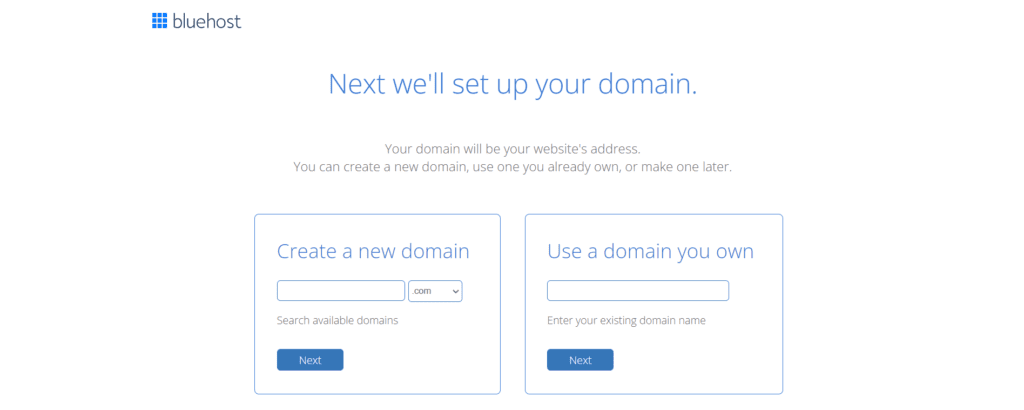The image depicts the homepage of Bluehost, a company dedicated to helping users create new websites or domains. The company's name, "Bluehost," is prominently displayed in the upper left-hand corner. The design is minimalistic, featuring a clean white and blue color scheme that adds to its modern appearance. Centered on the page is the instruction: "Next, we'll set up your domain. Your domain will be your website's address. You can create a new domain, use one you already own, or make one later."

Beneath this text, users are given two options, each accompanied by a clickable button to proceed to the next step. The first option, "Create a New Domain," includes a dropdown menu next to the input field, allowing users to select different domain extensions such as .com. There is also a "Search Available Domains" function to ensure the chosen name is unique and available. The second option, "Use a Domain You Own," provides an input field for users to type in their existing domain, enabling them to continue with customizing an already-owned address.

These two options, either creating a new domain or using an existing one, are the only available actions on this page, guiding users through the initial steps of setting up their website.